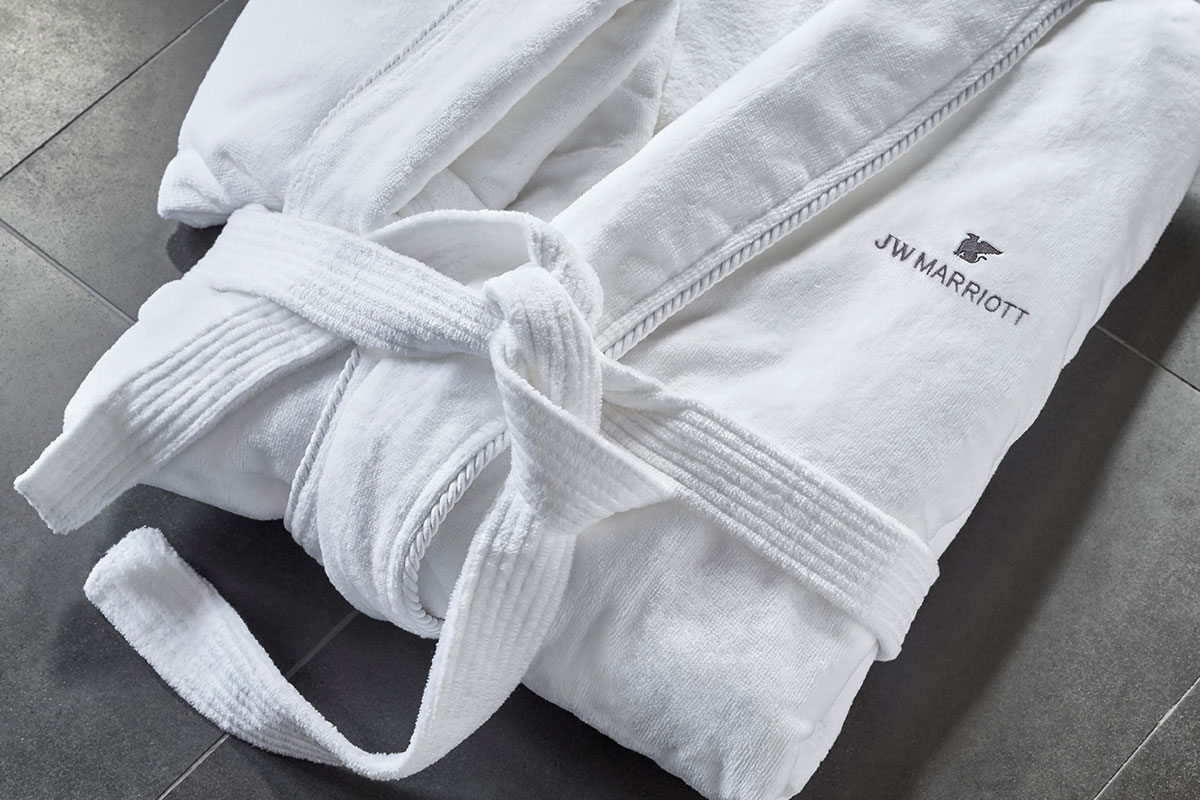This photograph features a meticulously folded, pristine white JW Marriott hotel robe, elegantly embroidered with the hotel's logo and name on the chest. The robe is staged on what appears to be a dark slate or gray tiled surface, which enhances the robe's crisp whiteness and high-quality fabric. The ribbed tie is already knotted and draped across the front, adding a touch of neatness and readiness. The well-lit, top-down perspective from about a 60-degree angle effectively showcases the luxuriousness of this amenity, making it perfect for use in stock photography, travel websites, or hotel promotional materials.